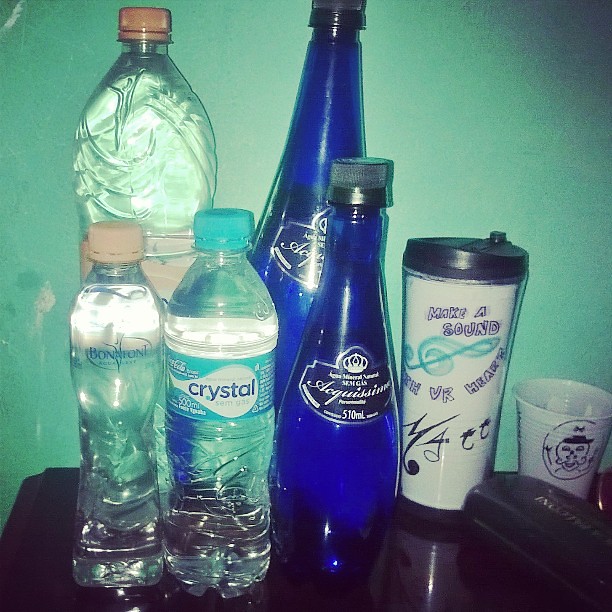On a brown wooden end table stands an eclectic collection of water bottles and cups. Dominating the scene are multiple bottles of various sizes and colors. Two slender blue glass bottles labeled "Aquazance" contrast with another delicate pink-capped, slender bottle marked "Bonfant." A Coca-Cola Crystal bottle with a blue lid is also distinctly visible. Among these is a customizable tall sippy cup, decorated with the phrase “make a sound with your heart” amidst musical notes. Beside it sits a quirky white plastic cup, common in hospital waiting rooms, featuring a hand-drawn face in black Sharpie. A small shot glass with a stick figure and the letter "N" adds an eccentric touch. To the bottom right, a glasses case subtly rests. The backdrop is a green wall marred by a large white stain on the left side, enhancing the overall visual intrigue of the table's contents.